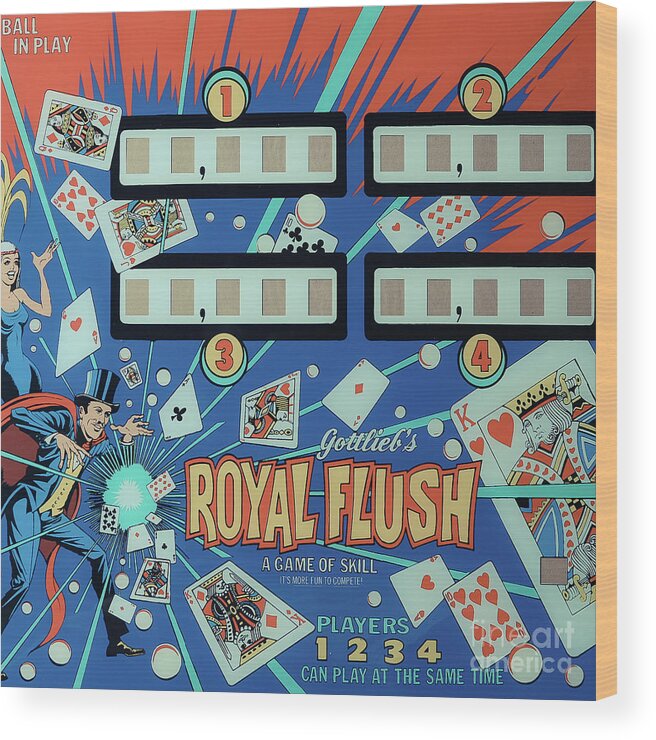The image depicts the box of a vintage game called "Gottlieb's Royal Flush," described as a game of skill that allows up to four players to compete simultaneously. The central theme revolves around a poker card variation, with a magician and his attractive female assistant prominently featured on the left side. The magician, dressed in a traditional top hat, suit, vest, and cape, appears to be conjuring cards in a dramatic display. The background is vividly colored, with a red explosion emanating from the magician and blue rays decorated with playing cards like the Ace of Hearts, Queen of Diamonds, Jack of Hearts, Ace of Clubs, Ace of Diamonds, King of Diamonds, and King of Hearts. Notably, the depiction includes two Ace of Hearts, indicating an intentional or unintentional duplicity within the set. The scene is complemented by blue lasers and marble shapes, enhancing the magical, mystical atmosphere. The design evokes an old-fashioned aesthetic, possibly from the mid-20th century, and includes scoring screens labeled 1, 2, 3, and 4, where players can track their cumulative scores. This detailed artwork suggests a blend of pinball mechanics and card game elements, emphasizing skill and competition to heighten the gaming experience.